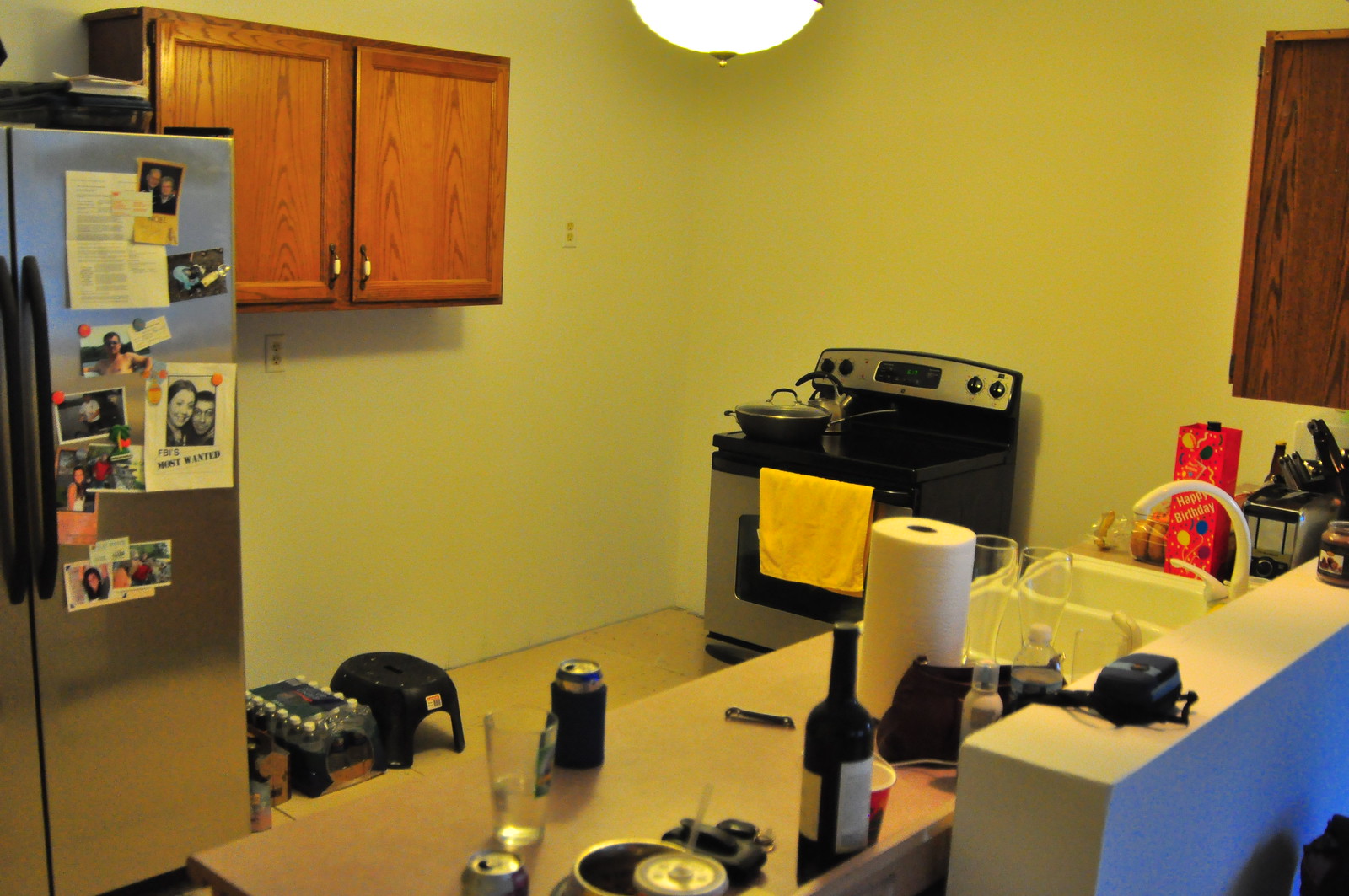This photograph captures an unusual and somewhat dimly lit kitchen interior. The walls of the kitchen are painted white, though the dim, yellow-toned lighting casts a warm filter over the entire scene, making the wall color appear ambiguous. The view focuses on the corner of the kitchen, revealing two intersecting walls. On the right wall, there is a window that has been boarded up with a dark wooden plank. In the corner, standing alone without any counters on either side, is a black and silver electric stove with a glass top. A frying pan with a lid rests on its surface.

On the left wall, a silver two-door refrigerator with black handles stands prominently. Its doors are adorned with various pictures and papers held up by magnets. Mounted on the wall above and to the right of the refrigerator are two wooden cabinets providing additional storage space.

In the foreground stands a kitchen island which has a white sink embedded in it. The island is cluttered with various items, contributing to the unusual and cluttered appearance of the space.